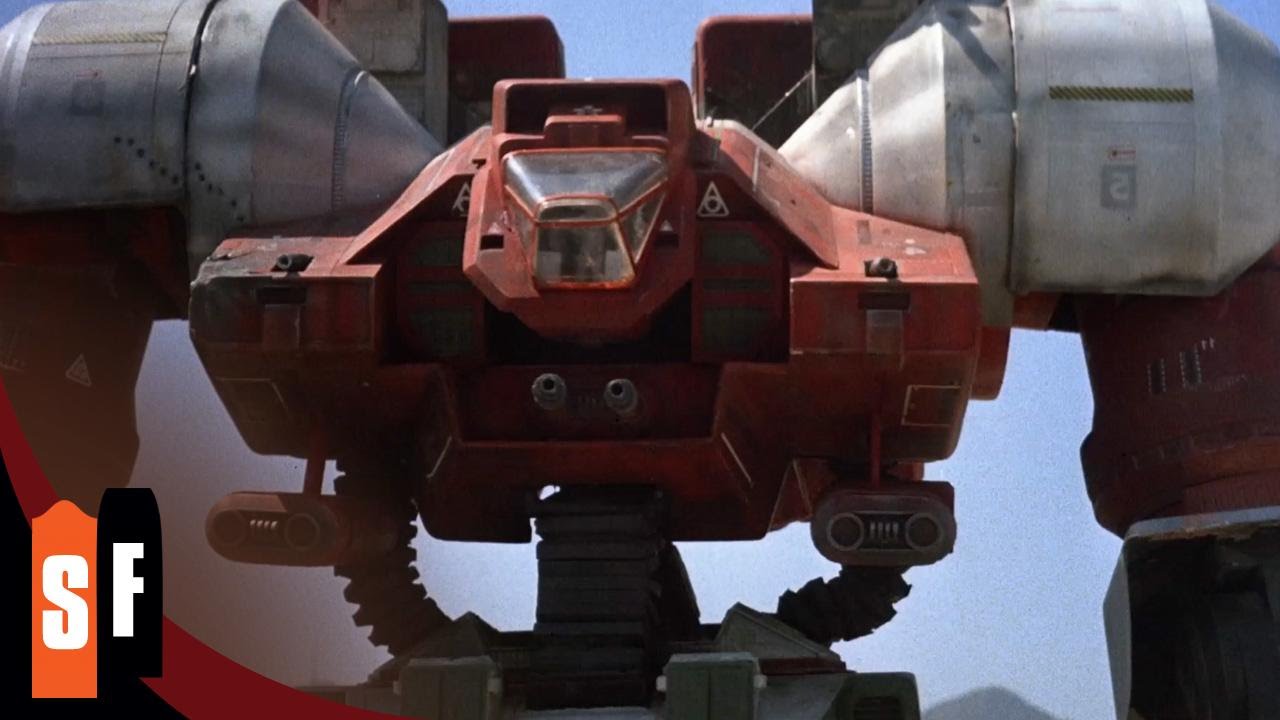This is a detailed, color screenshot of a large, bulky robotic machine that resembles a Transformer, potentially taken from a movie scene. The robot's main body is predominantly red, while its large, cylindrical shoulders are silver. The visible parts of its arms are also red, extending only up to the elbow. The robot's head appears to be a glass cockpit at the center of the chest, surrounded by red metal. The cockpit is flanked on either side by large, cylindrical containers, one of which features a mirrored number "5" with a small arrow pointing towards the cockpit. The robot’s spine is black, with support ridges curving from each side, suggesting it can tilt side to side. At the front of the machine are multiple turret guns: two barrels on each side, two more in the very center, and a gun mounted on each shoulder. In the bottom left corner, there is a logo comprising the letters 'S' and 'F' in white; 'S' is set against an orange bookmark-shaped background, and 'F' against a black bookmark-shaped background. This logo is accompanied by red and black swoops making an appearance in the corner.